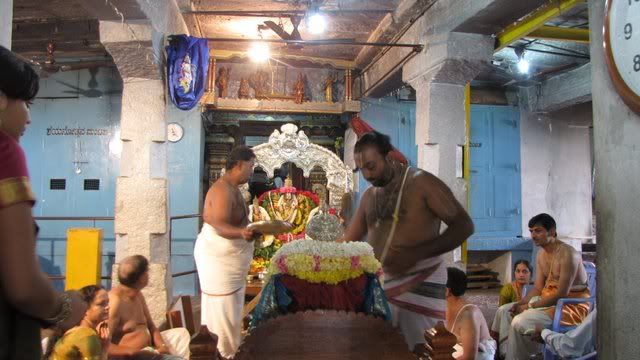The image depicts an indoor scene inside what appears to be an older, possibly Asian or Indian-style building, featuring white columns and an ornate ceremonial setup. In the center, two shirtless men, clad in white wraps around their waists, stand on either side of a central figure, which could be a statue or an individual adorned with a sparkly silver hat and robe, likely part of a religious or ceremonial event. Surrounding them are several onlookers—some seated on the ground and others on blue chairs. Notable details include a woman dressed in traditional Indian attire on the far left, and another woman in a yellow outfit sitting beside a white pillar. On the right, there's a portion of a clock displaying the numbers 8 and 9, hinting at the passage of time within this scene. The room also features stone or concrete walls, blue shelves or cabinets in the background, and a white banner with "Protect Your Memories for Less" alongside the "PhotoBucket" watermark obscuring parts of the picture.